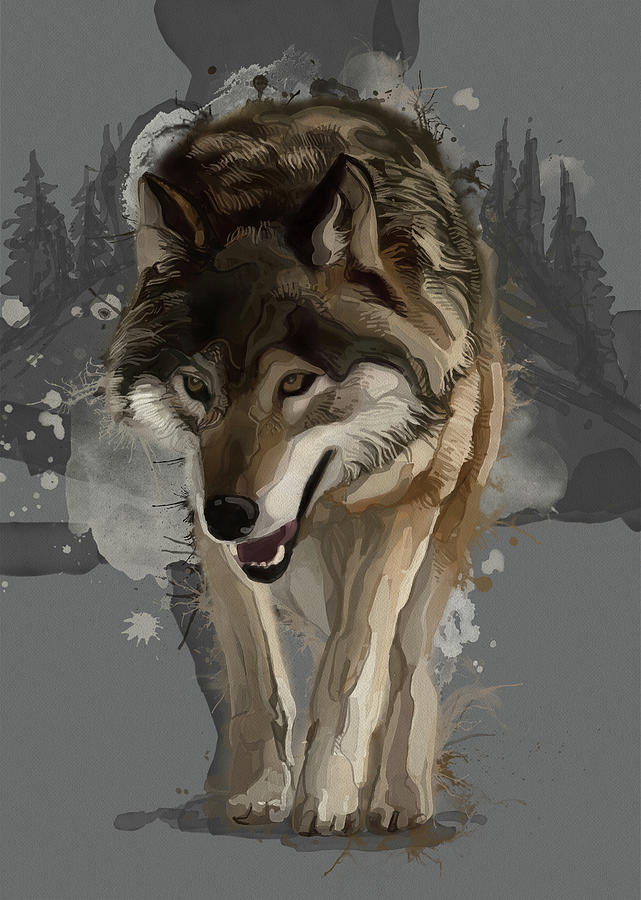The image depicts a wolf with a serious facial expression, showcasing unkempt brownish-gray fur with lighter shades around its mouth and nose. The wolf has an open mouth, revealing its teeth, and a black nose. The backdrop features a gray, cloud-filled sky over a snowy, mountainous landscape. Scattered across the scene are dark trees, resembling either pines or palms, casting shadowy silhouettes. The overall environment exudes a wintry, desolate vibe with predominant colors being shades of gray, white, black, and various browns. The illustration style appears somewhat rough and sketch-like, possibly created with alcohol markers or a similar medium, lending a less detailed, more artistic aesthetic to the image. There is no visible text in this evocative portrayal of the wolf subtly walking away from the forest.